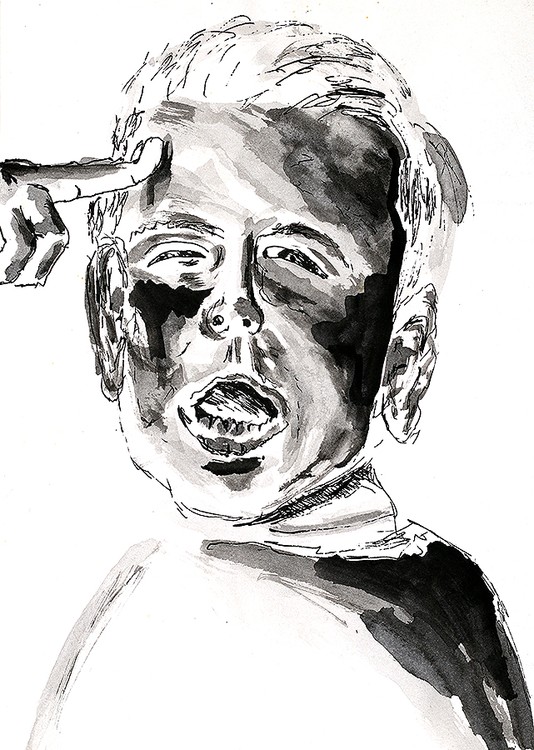The image depicts a black and white drawing of a man's face facing forward, created with a mix of ink and watercolor. The background is entirely white. The man's hair, which is ear-length and appears light in color, contrasts against the monochrome tones used in the portrait. His forehead is predominantly gray, with a darker shade on the right side. His eyes are half-closed, with dark shading under both eyes and on his left cheek, while the right cheek is mostly gray. The man's mouth is open, showing a thin upper lip and a thicker lower lip, with a bit of black shading beneath it. Details of his nose include small black dots for the nostrils and a gray area above the right nostril. 

Positioned on the left edge of the image is a hand, with an index finger pressing against the man's right temple, and two more fingers partially visible and folded. The man's neck is partially visible, with some black and dark gray shading on the right side, extending into what appears to be some form of clothing. While only a small portion of his chest and shoulders is visible before the drawing fades off at the bottom, the middle section beneath his head is left white, accentuating the detailed shading on his face. The ears, which are quite prominent, add to the character of the portrait, giving a realistic yet slightly exaggerated expression as if captured in a candid, less flattering moment.